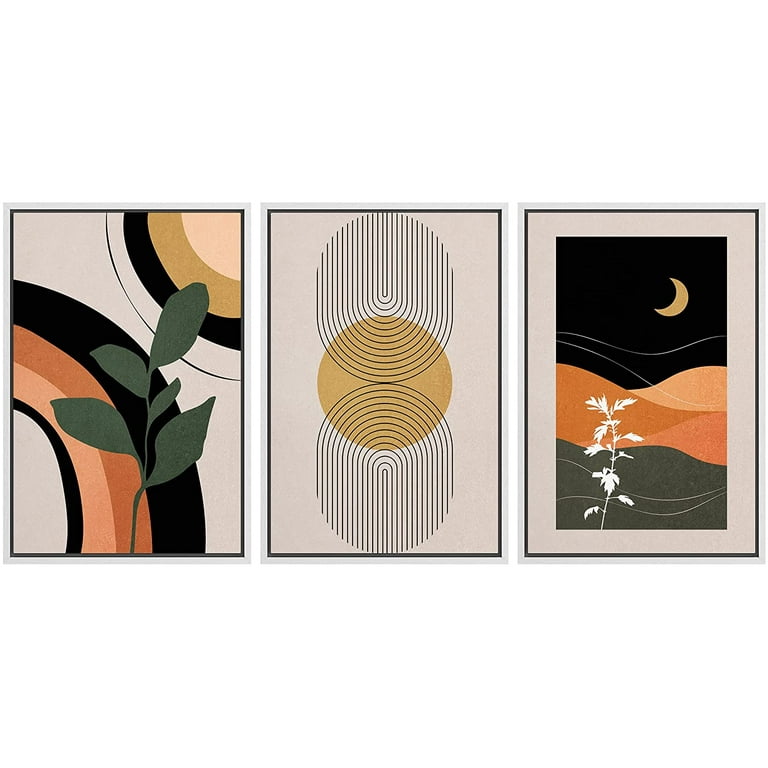This image displays a vibrant tryptic artwork, each piece rectangular and slightly taller than wide, all framed with a white border and set against a light khaki or taupe background.

The left panel features an arrangement of layered half-circles in varying sizes and colors—ranging from beige, black, peach, to orange—giving a cascading, sun-like effect. These shapes are partly obscured by a stylized, dark green plant with large leaves, adding a touch of natural intrigue against the semi-abstract backdrop.

In the minimalist middle panel, two black, fingerprint-like curves expand from a small thin line into larger, circular arcs, intersected by an opaque orange circle that stands out against the beige background. This central design evokes a sense of simplicity and symmetry, framed by the subtle, continuous lines.

The right panel portrays a serene night scene with a yellow crescent moon hanging over a series of cascading hills. These hills transition in color from black at the top to peach, orange, pink, and olive green, each demarcated by white lines. A white, silhouette plant extends upwards, adding a delicate contrast to the darker hues, completing the harmonious composition.

Each piece of the tryptic art is meticulously detailed, blending geometric forms with organic elements to create a cohesive, visually engaging triptych.